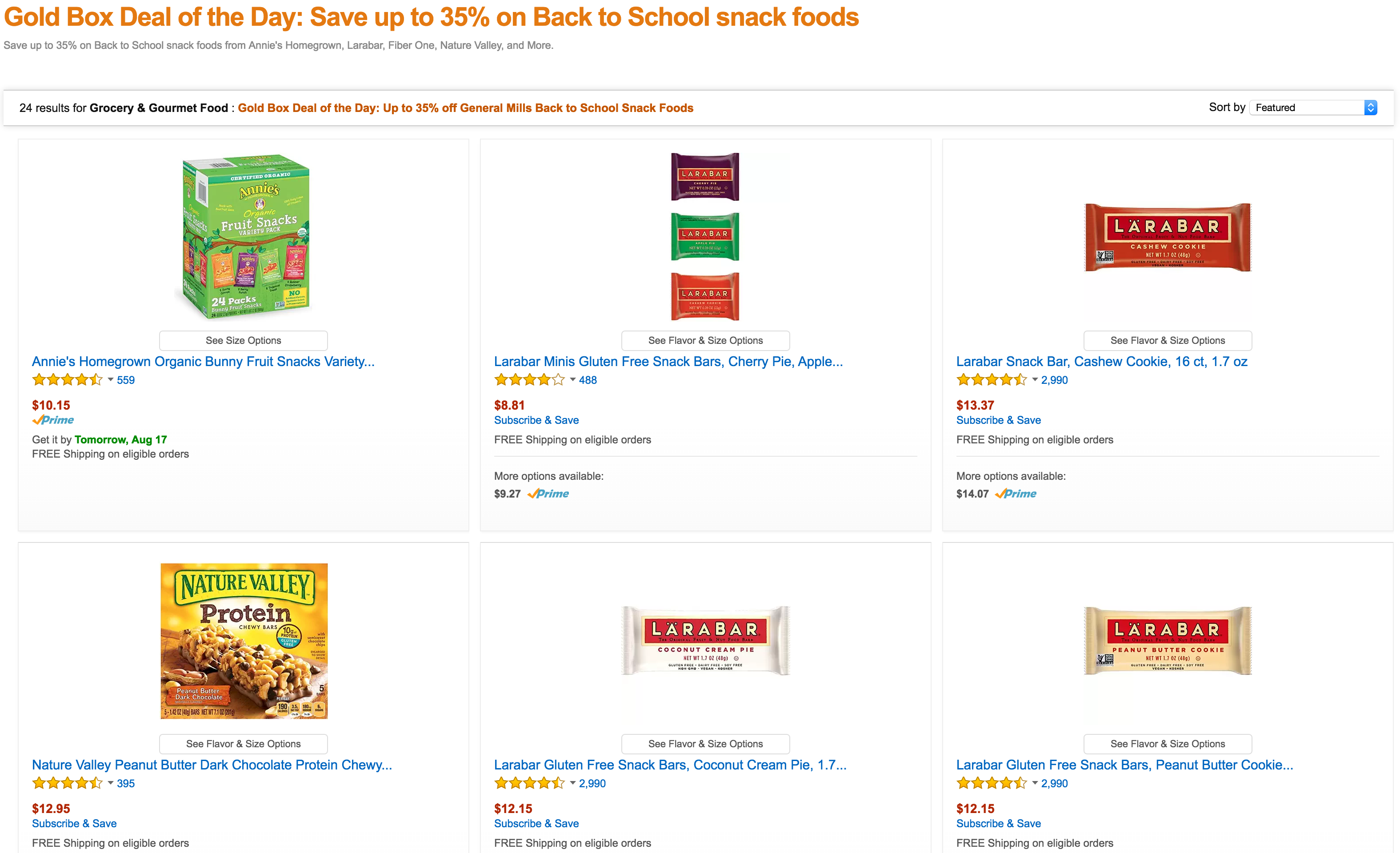The image showcases a screenshot of an Amazon webpage featuring a "Gold Box Deal of the Day" promotion. Dominating the top left corner is an orange text announcing significant savings: "Save up to 35% on back-to-school snack foods." Directly beneath this, in a slightly transparent gray text, the offer details: "Save up to 35% on back-to-school snacks from Annie's Homegrown, Lara Bar, Fiber One, Nature Valley, and more." This clearly positions the promotion as catering largely to healthier snack options. 

Displayed below the promotional text are sorted search results for "Grocery and Gourmet Food," highlighting a collection of snack products available at a discounted rate. The layout consists of two rows, each containing three products. Here are the six items presented:

1. **Annie's Homegrown Organic Bunny Fruit Snacks** - Positioned at the top left, these organic fruit snacks are a popular choice for kids.
2. **Lara Bar Minis Gluten-Free Snack Bars** - Available in flavors like Cherry Pie, Apple, and others, they are the middle item in the first row.
3. **Lara Bar Snack Bar Cashew Cookie** - The last item in the first row, this bar is known for its simple, wholesome ingredients.
4. **Nature Valley Protein Peanut Butter Bars and Peanut Butter Dark Chocolate** - The first item in the second row, these bars provide a protein-rich snack option.
5. **Lara Bar Gluten-Free Coconut Cream Pie** - This item, located in the middle of the second row, offers a taste of coconut in a gluten-free format.
6. **Lara Bar Gluten-Free Peanut Butter Cookie** - The final item, combining the simple taste of peanuts into a gluten-free snack bar.

Several of these products are labeled with the "Prime" badge, reinforcing that the website is Amazon and indicating that these items are eligible for Prime benefits.